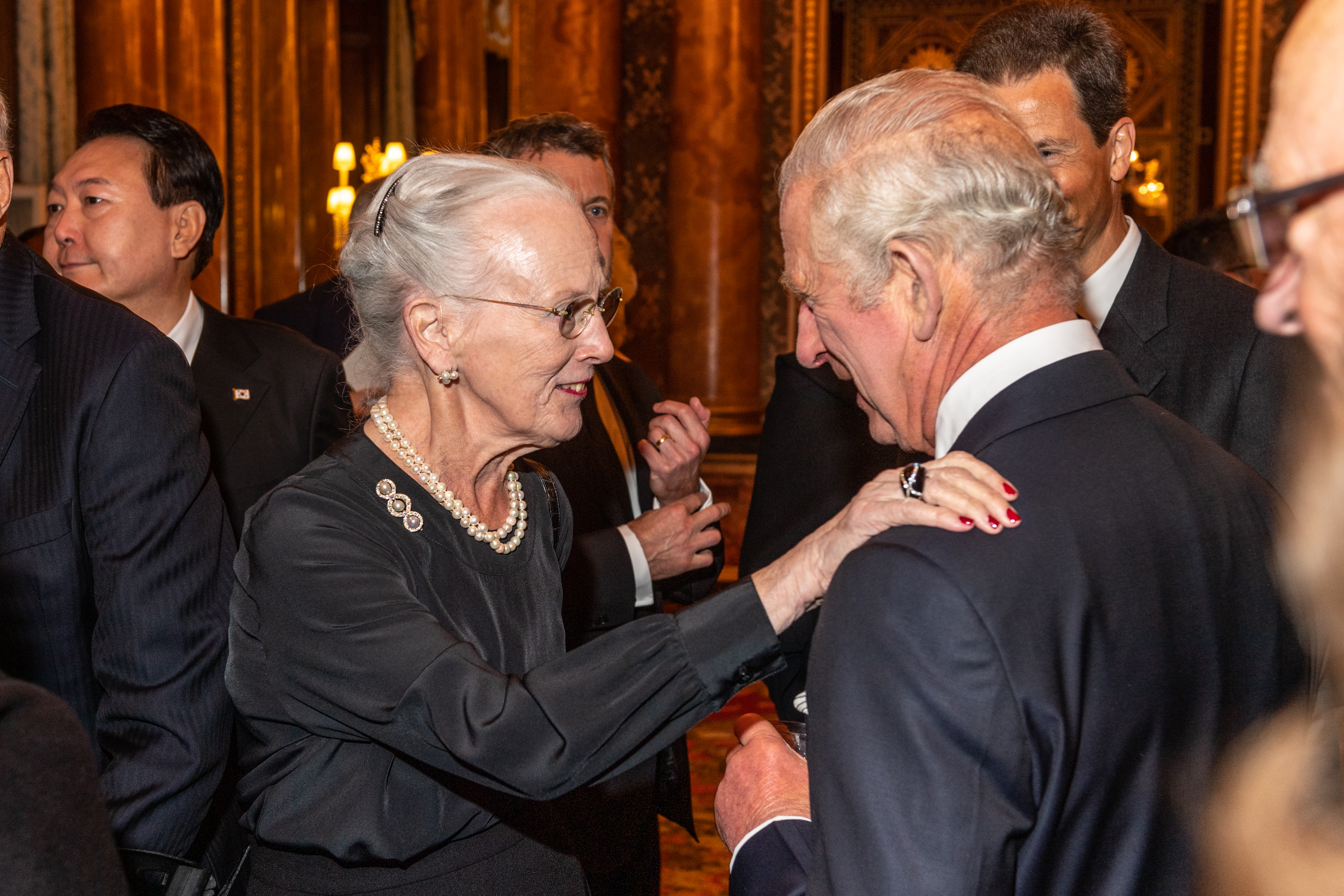This photograph captures an elegant moment between King Charles and an older woman, surrounded by a crowd of people in an opulent setting. King Charles, identifiable by his gray hair combed over a balding back, wears a dark-colored suit and a white collared shirt. He is smiling warmly. The elderly woman, clad in a black dress, sports a black ring with diamonds on her right hand, which she has placed on King Charles' left shoulder. Her hair is neatly combed back into a low bun, and she is adorned with glasses, a beaded pearl necklace, pearl earrings, and red lipstick. She too is smiling, though more subtly compared to King Charles. The background is luxurious, hinting at an upper-class venue with a golden, castle-like or church-like interior. Several other figures, including an Asian man in a suit, are present in the scene, contributing to the formal and refined atmosphere.